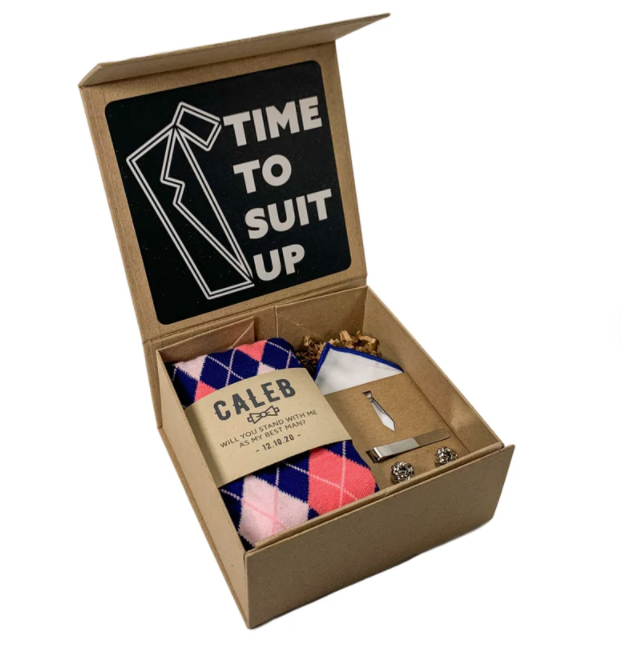The photograph depicts an open, heavy-duty cardboard gift box against a white background. The box is brown with a flip-open lid. On the inside of the lid, a black square features white lettering that reads "Time to Suit Up," accompanied by a graphic of a person in a suit. Inside the box, on the left-hand side, there's a folded Argyle sweater in blue and different shades of pink, wrapped with a brown label that says "Caleb" and displays an image of a bow tie. The label includes the message, "Will you stand with me as my best man, 12-19-2020." To the right of the sweater lie a couple of cufflinks, a tie clip, and a neatly folded tie or possibly a shirt. The pocket square, which is white with blue edges, completes the ensemble.